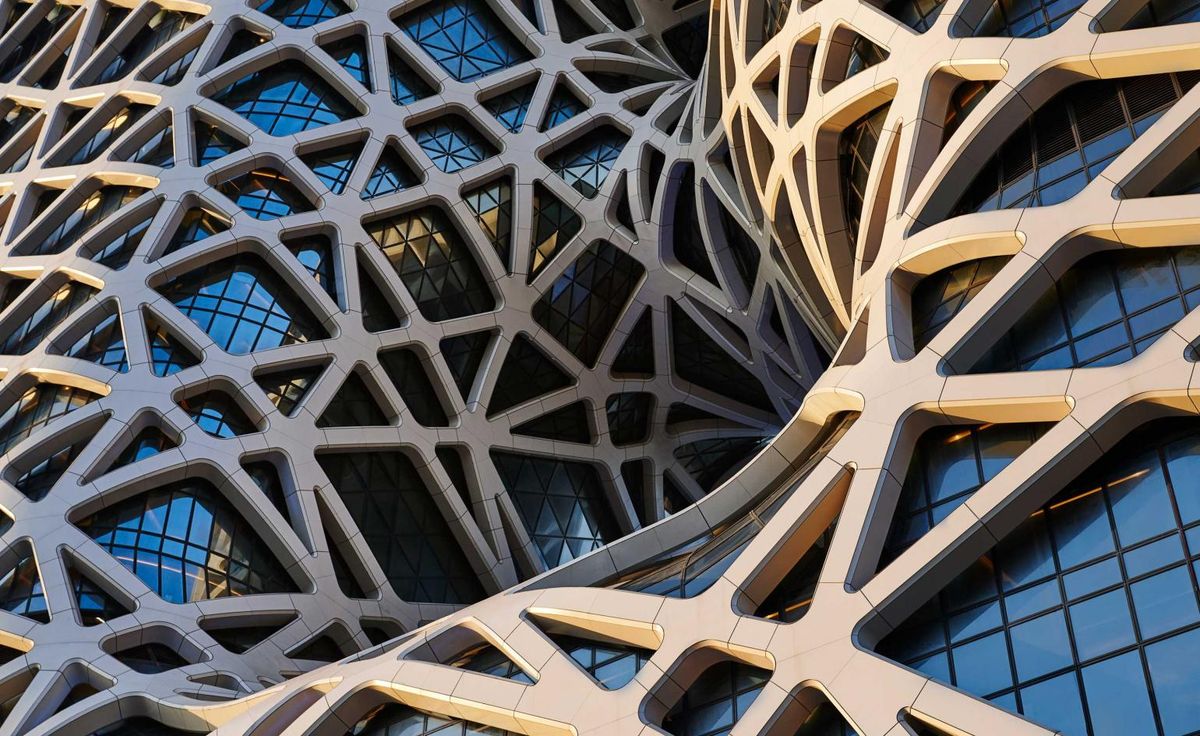The image depicts a striking piece of modern architecture that merges an intricate, lattice-like metal exoskeleton with a tall office building. This lattice, resembling a complex network of atoms or interlinked bones, exhibits a smooth, welded structure with a mix of triangular and square patterns. The metal framework starts lighter on the left, transitions to darker gray in the center, and lightens again on the right side, creating a dynamic gradient effect. 

Behind this elaborate metalwork is a backdrop of blue-tinted glass, segmented with black lines forming variously sized squares and rectangles, reminiscent of window panes. The central part of the structure dips inward, evoking the image of being sucked into a black hole, casting shadows and enhancing the three-dimensional illusion. Light plays across the surface, illuminating sections in a gradient from the left and right, while the middle remains more shaded. The overall effect is a detailed and visually compelling blend of geometry and modern design.